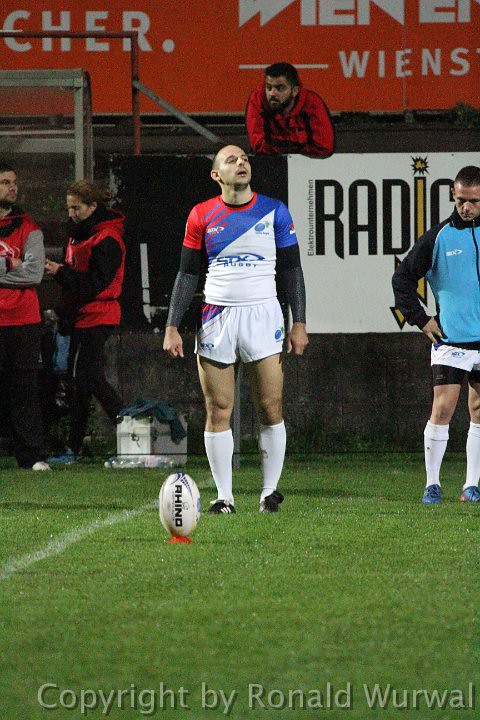This grainy photograph, attributed to Ronald Werwal, captures a moment on a green field during what appears to be a rugby match, given the ball’s shape and its placement on a red tee. The primary focus is on two players: the central figure is a balding man preparing to kick the ball. He’s wearing a distinctive red, blue, and white jersey with black sleeves, white shorts, and white leggings, and is looking to his left. To the right edge of the image stands another player in a powder blue top with black sleeves, white and black striped shorts, white leggings, and blue shoes. The field features scattered spectators or officials in red jackets, possibly groundskeepers, and there's a partially visible banner that says "radio..." in the background. The image concludes with a "copyright by Ronald Werwal" watermark at the bottom edge.